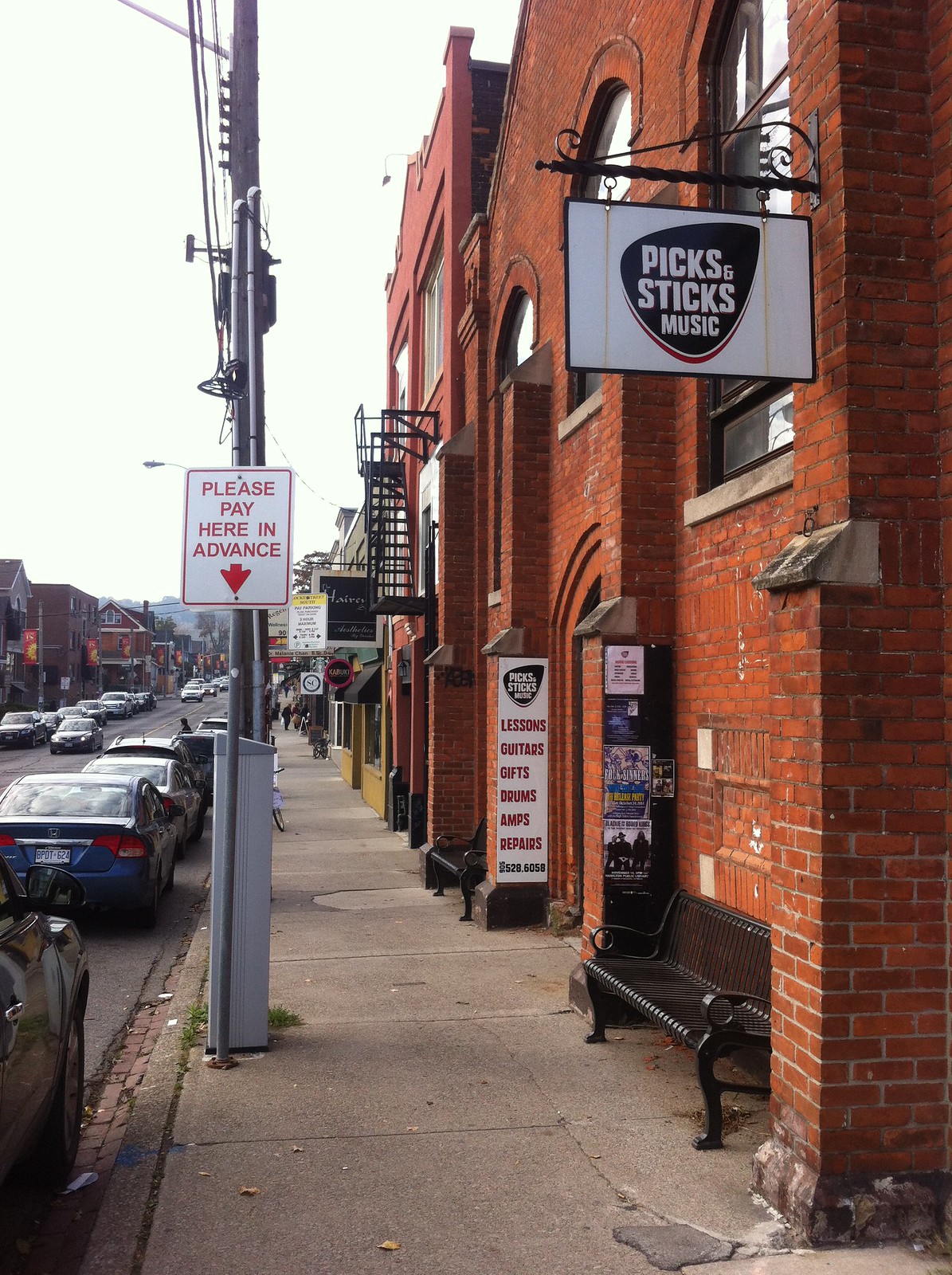This is a detailed photograph of a bustling city street captured in front of a music store named Picks and Sticks Music. The scene is set on a lively city block that features brick buildings reminiscent of small towns in Georgia. The Picks and Sticks store is prominently highlighted, with its eye-catching signage shaped like a guitar pick, displaying the store's name against a white background with a black border. There are additional advertisements for the store visible in the distance, listing services such as lessons, guitars, gifts, drums, amps, and repairs, although some details are slightly blurry.

Nearby, a parking pay machine stands with a clear sign instructing, "Please pay here in advance.” The street is lined with benches where passersby can rest, and numerous other stores line the block, inviting exploration further down the road. The sidewalks are clear, but the streets are quite busy, with numerous cars both parked and in motion, suggesting a vibrant, possibly downtown, area. People can be seen walking along the sidewalks, reinforcing the sense of a lively, active city setting.